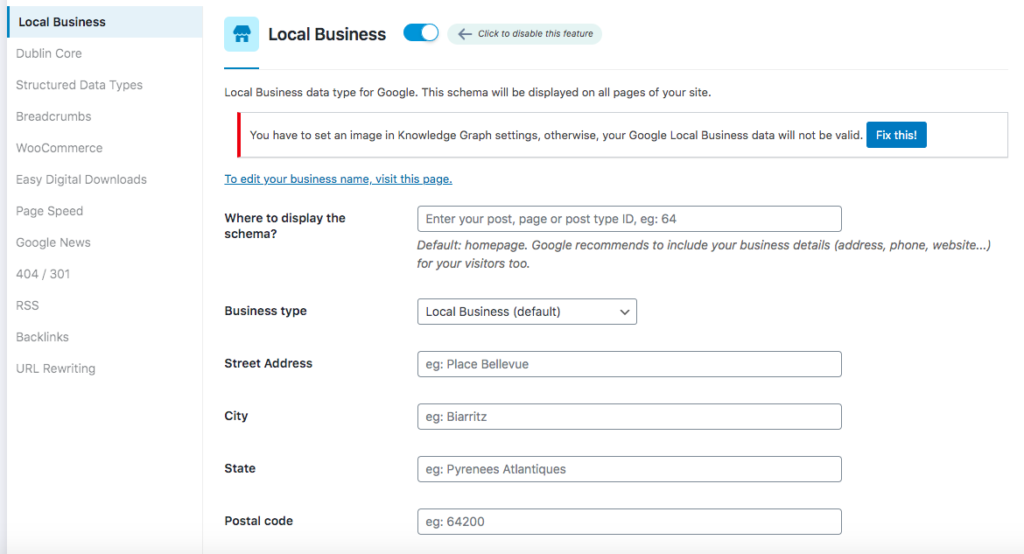**Caption:**

This is a detailed screenshot of a website interface, showcasing a multitude of clickable options on the left-hand sidebar, including "Local Business"—the page currently displayed. The sidebar also lists various other categories such as Dublin Core, Structured Data Types, Breadcrumbs, WooCommerce, Easy Digital Downloads, PageSpeed, Google News, 404-301, RSS, Backlinks, and URL Rewriting.

In the "Local Business" section, a toggle switch is set to the "on" position, accompanied by an option to disable this feature. Below this toggle, there's descriptive text explaining that the local business schema data type for Google will be displayed across all business pages of the website. A notification prompts users to set an image in the knowledge graph settings, warning that failure to do so will invalidate the Google Local Business data. A blue button labeled "Fix This" is provided for immediate action.

Further down, a hyperlink in blue text allows users to edit their business name by visiting a specified page. The interface also includes a section for filling out detailed information about the business, such as where to display the schema, and entering the post, page, or post type ID (e.g., 64). Additionally, it offers fields to input business details, including business type, street address, city, state, and postal code, with a recommendation from Google to include these details on the default home page.